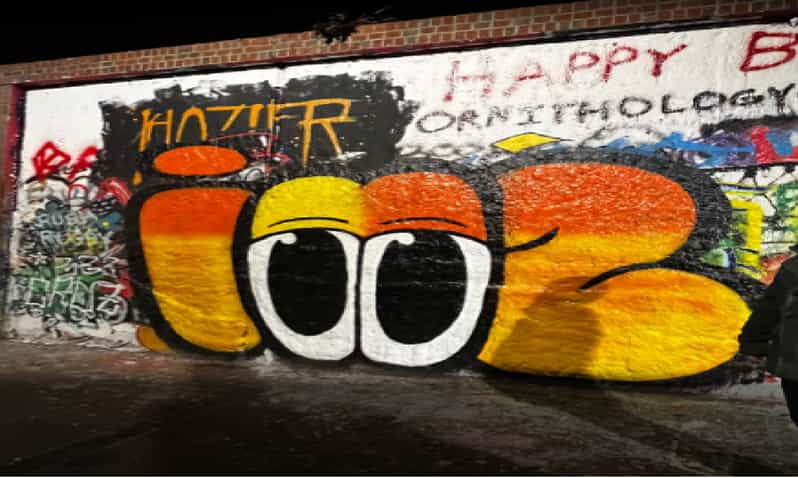This photograph captures a vibrant graffiti mural that spans the side of a red brick building, taken at night. The mural, set against a white background, predominantly features a creatively designed central motif. In the middle, there are two large eyes with eyelids that could also be interpreted as the letter "O." To the left of these eyes, there is a smaller eye with a dot at the top, and to the right, what appears to be a heavily stylized number "2" or perhaps the letter "Z," all portrayed in candy corn colors of orange, yellow, white, and outlined in thick black lines.

Above this central artwork, the words "Happy Birthday Ornithology" are prominently displayed in red and black letters. To the left, on a black background with yellow letters, the name "Hozier" is written. The mural is a mix of various other graffiti elements in reds, blacks, blues, whites, and greens, suggesting multiple layers of tagging over time. In the bottom right of the image, the arm and part of the torso of a person are partially visible, standing on a plain, brick-colored sidewalk in front of the mural.